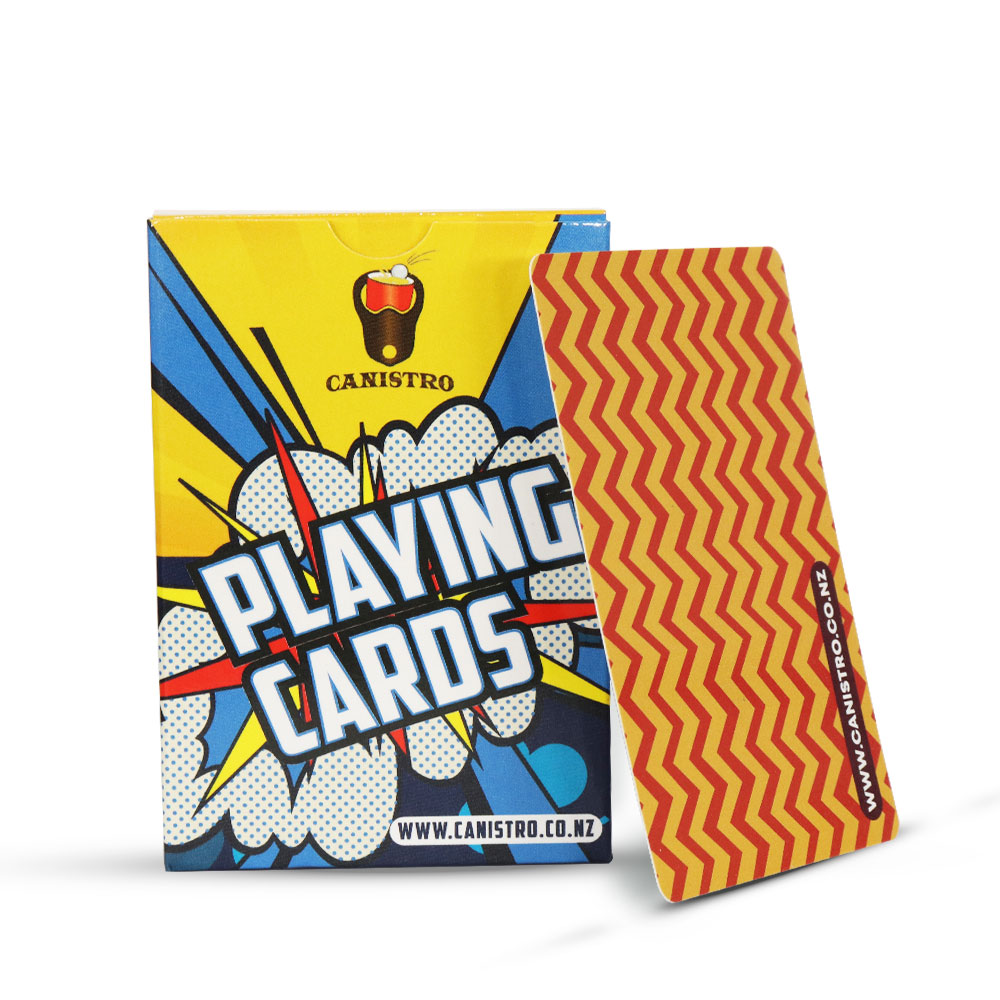A detailed image of a pack of playing cards is set against a plain white background. The main focus is a rectangular, thin box with vibrant design elements. Dominantly yellow and blue, the box prominently features the words "PLAYING CARDS" in large, white, all-caps block letters outlined in black, printed diagonally across the center. Surrounding the text is an explosion pattern with sharp, triangular points in red, yellow, and blue colors emanating outwards. 

A distinctive white cloud with a black border is positioned in the middle of the box, filled with a checkerboard pattern of grey dots. The backdrop of the box is a mix of yellows and various shades of blue, forming a burst effect around the cloud. At the top of the box, a logo depicts a simplified red and brown mouse head wearing sun shades, detailed with a yellow nose and white hair, likely indicative of a 1950s revivalist style. Below the logo, in black uppercase font, is the brand name "CONISTRO."

Leaning against the right edge of the box is an individual card, its back featuring a bold, alternating zigzag pattern in red and yellow. In the lower right corner of the box and the lower left corner of the individual card, the website "www.conistro.co.nz" is displayed in white, capital letters against a black banner, indicating the card's origin.